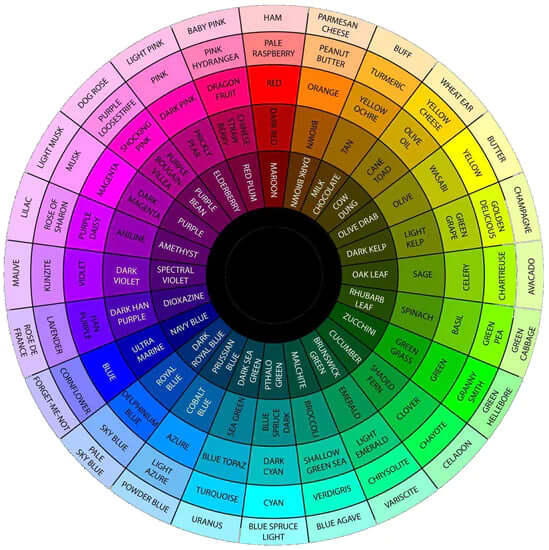This detailed image features a concentric circular chart where each ring is divided into color-labeled segments. At the center lies a black circle around which the first ring contains shades like maroon, dark brown, and other muted tones such as olive drab and dark kelp. The intricate design extends outward through five rings, each segmented by color and labeled accordingly. The arrangement puts darker colors predominantly on the left side and lighter ones on the right. The top of the wheel showcases shades of red, pink, and orange, transitioning to yellows and greens to the right. Toward the bottom, the chart presents blues, while the left side encompasses purples and darker blues. Each section within the rings has specific names for the colors and hues ranging from "peanut butter" and "pale raspberry" to "sage" and "light emerald," blending creative and botanical names. The entire chart visually progresses from dark at the center to more varied and lighter hues at the perimeter.